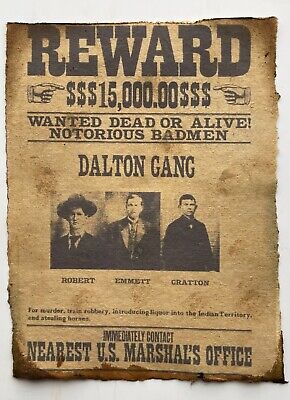This is a photo of an old, weathered Wanted poster that commands a reward of $15,000 for the capture of the notorious Dalton Gang, dead or alive. The poster features three black-and-white headshots of the gang members, identified as Robert, Emmett, and Grattan, who appear to be white males, clean-shaven, with one wearing a hat and all dressed in suits. The poster, which has a sepia-tone coloration and is printed on aged, scroll-like paper with frayed and stained edges, evokes the atmosphere of the Wild West. Two hands are pointing at the reward amount to emphasize its significance. Instructions at the bottom urge anyone with information to "immediately contact the nearest U.S. Marshals Office." The overall condition and design of the poster give it an authentic feel, suggesting it could be a legitimate piece from the late 1800s.